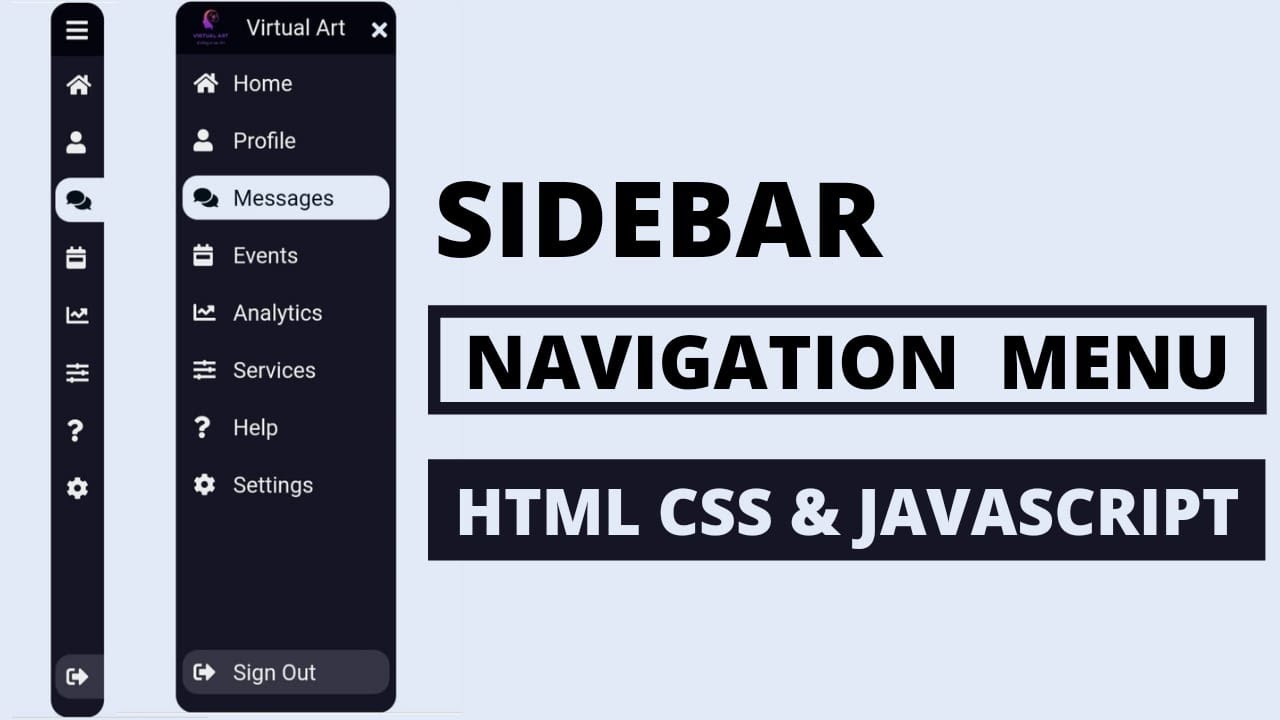The image, captured from a smart device, presents a left-to-right horizontal layout with a solid, flat, bluish-gray background devoid of texture or dimension. Along the left-hand side of the image is a black, rounded, thin rectangular box containing several icons arranged vertically: three horizontal lines, a house icon, a person icon, a chat messages icon (highlighted), a calendar icon, an analytics services icon, and a question mark icon for settings.

Adjacent to this thin black box is a slightly broader rectangular section labeled "Virtual Art." This section provides a textual representation of the icons found in the previous box, with labels reading: Home, Profile, Messages (the current selection), Events, Analytics Services, Help, Settings, and a Sign Out button located at the bottom.

In the main portion of the image, on the flat bluish-gray background, there are large, bold, uppercase black letters spelling "SIDEBAR." Below this, encapsulated in a box, are the words "Navigation Menu," and beneath that, a black box with white text lists "HTML, CSS, and JavaScript."